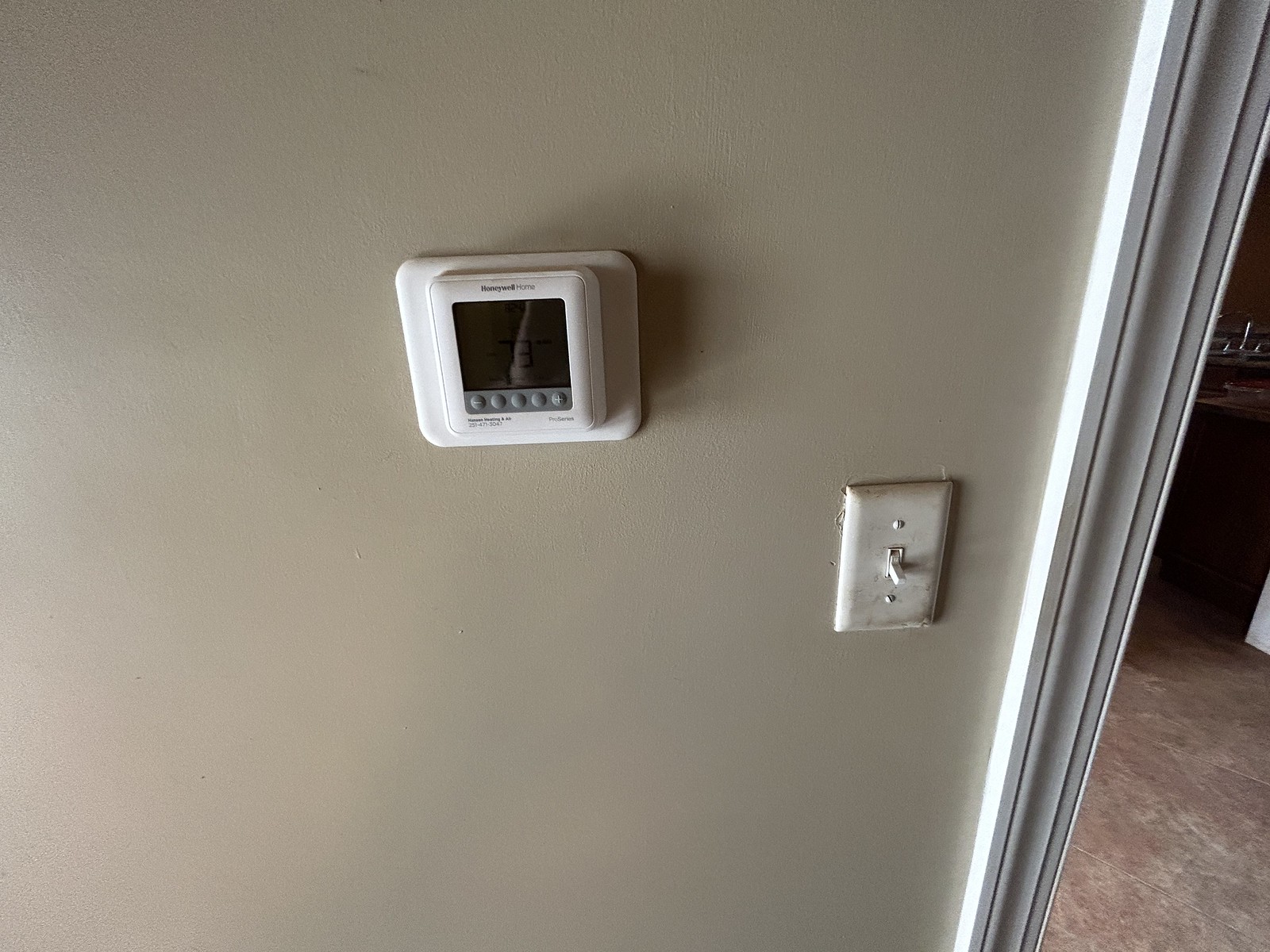The photograph captures a serene, albeit mundane, corner of a home interior. At the heart of the image is a plain white or beige-colored wall, subtly textured with an eggshell finish. Centrally mounted on this wall is a white Honeywell Home air conditioning control unit. Though the screen is dim, one can faintly discern the temperature setting, which reads 73 degrees. Below the screen, several circular buttons, including a plus and minus sign, provide temperature control options. 

Just down and to the right of the thermostat, a slightly dirty, well-used light switch is mounted. This traditional switch, clearly showing signs of wear and tear, resides next to some pristine white crown molding that delineates the border of a door frame. In the bottom right-hand corner of the image, a glimpse into an adjoining room reveals a section of tile flooring, adding a sense of depth and continuity to the scene.